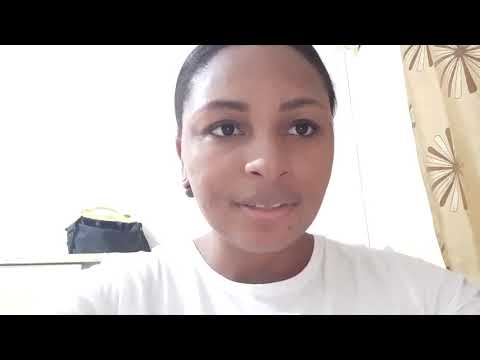The image depicts a young black woman from the shoulders up, wearing a white t-shirt. She has short black hair and a distinct gap between her front teeth, with her mouth slightly open, adding a hint of a smile to her expression. A dark mole is noticeable near her chin. The room is bathed in bright light, making the predominantly white background appear even more luminous. To the right of the woman hangs a light tan curtain featuring brown and white flower or star-shaped decorative patterns. On the left side of the image, there is a thin white shelf holding a black purse with yellow straps. Additionally, a black strip runs horizontally across the top and bottom of the image, framing the scene.